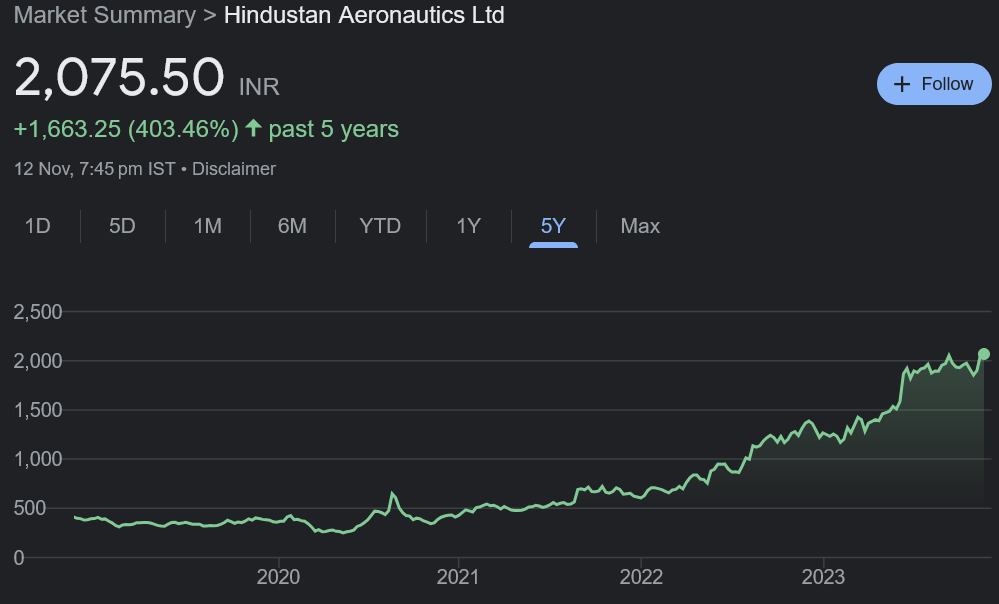The image is a screenshot of a graph with a gray background. In the upper left corner, it reads "Market Summary," followed by a small arrow pointing to the text "Hindustan Aeronautics Ltd." Directly below this, in large white font, the current value of "175.50 INR" is displayed. On the far right, there is a blue oval with black text that says "Follow."

On the next line, the text shows a value of "+1,663.25." While the currency is uncertain, it might not be dollars. This value is followed by open parentheses showing "403.46%" with a small upward-pointing arrow beside it, accompanying the text "Past 5 years."

Below this, in small gray font, it reads "12 November, 7:45 PM IST" followed by the word "Disclaimer." Underneath, there is a chart labeled at the top with various time frames: 1D, 5D, 1M, 6M, YTD, 1Y, 5Y, and MAX. The "5Y" option is selected, indicated by a blue underline below it. The graph itself is displayed below these labels, with a vertical scale on the left side ranging from 0 to 2,500.